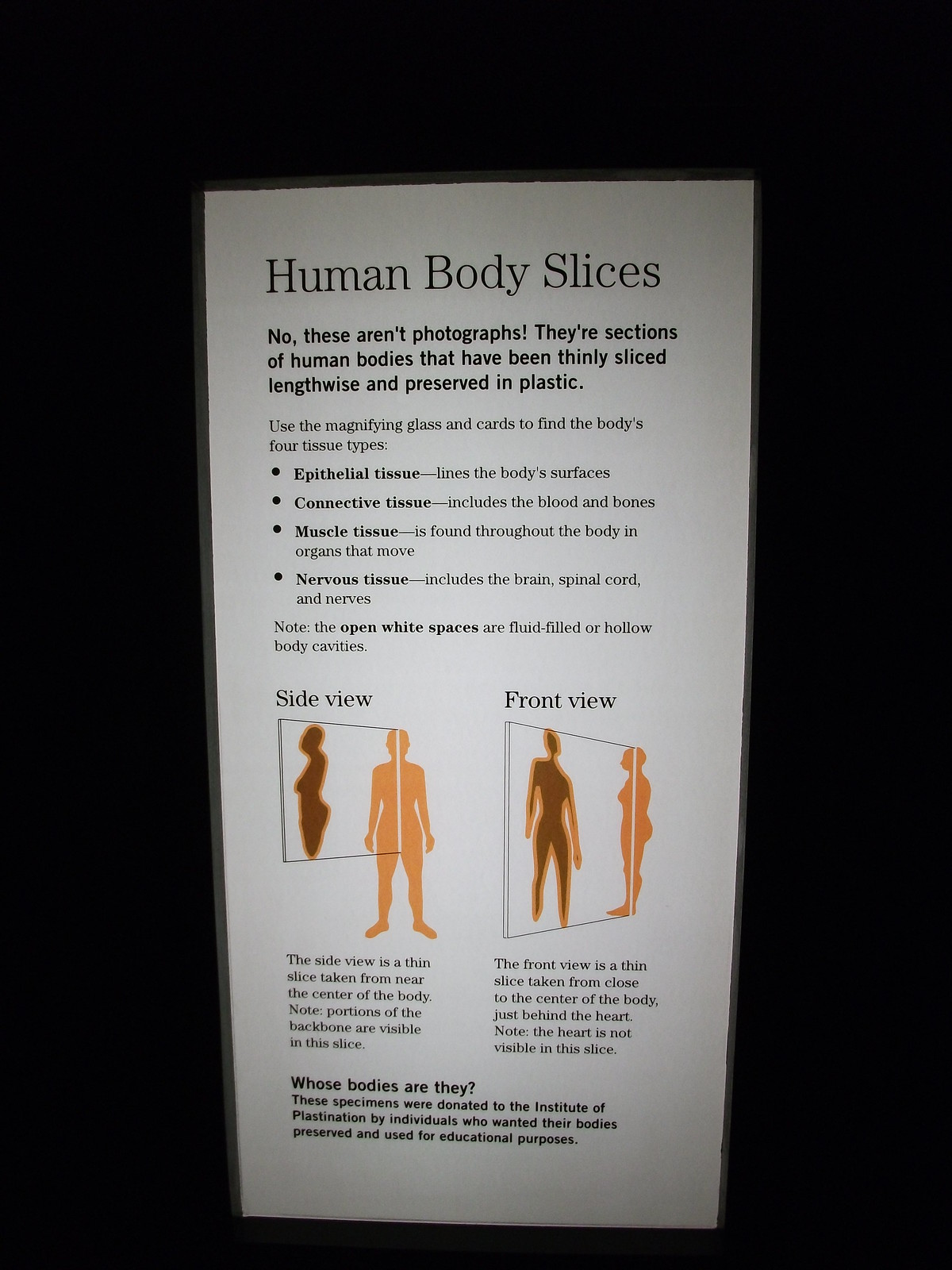The image showcases an instructional panel against a black backdrop that focuses on the concept of "human body slices." The white sheet at the forefront details various educational aspects related to the subject. The heading, "Human Body Slices," is prominently displayed in a large font at the top.

The text explains that the slices depicted are not photographs but actual sections of human bodies that have been thinly sliced lengthwise and preserved in plastic. It instructs viewers to use a magnifying glass and cards to identify four types of body tissues: epithelial, connective, muscle, and nervous tissue. The panel also notes that open white spaces in the slices represent fluid-filled or hollow body cavities.

Beneath this information, the sheet contains illustrative diagrams of a human body from both side and front views, rendered in shades of orange and brown. At the bottom, a section titled "Whose bodies are they?" reveals that the specimens were donated to the Institute of Plastination by individuals who wished to have their bodies preserved for educational purposes. All text on the sheet is in black, standing out clearly against the white background.